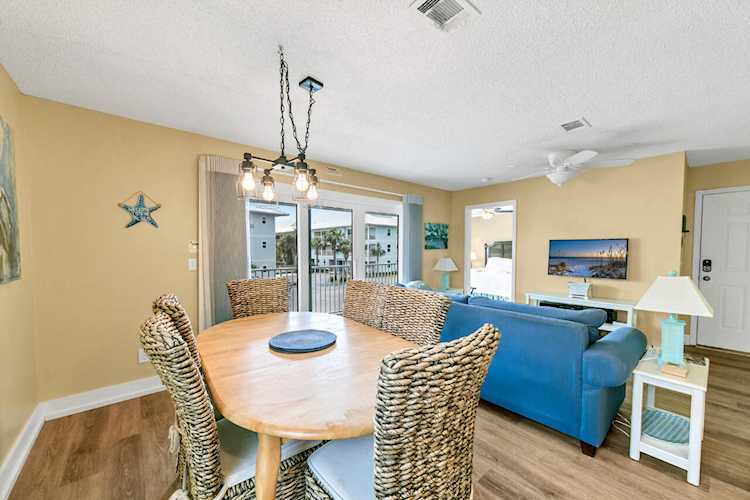The vibrant color photograph captures the interior of a home, showcasing a dining and living room in a harmonious open-plan layout. The floor is covered with light-colored wooden planks that add warmth to the space. Central to the image is a round wooden dining table, featuring a black circular centerpiece. The table is surrounded by several rattan-style chairs with plush white cushions, creating a cozy dining experience. 

Above the dining table hangs a modern lighting fixture with four bulbs, creating a soft glow that enhances the room's ambiance. The walls are painted a cheerful yellow, and a decorative starfish hangs prominently, adding a touch of seaside charm.

A large sliding glass door provides a view of an adjacent apartment building and numerous swaying palm trees, bringing an element of the outdoors inside. In the living area, a large blue couch offers comfortable seating, complemented by a small white side table adorned with a lamp featuring a turquoise base and a white shade. 

A sleek white ceiling fan hangs above, ensuring a comfortable temperature year-round. A flat-screen TV is mounted above a white console table, displaying a serene ocean scene that adds to the coastal theme of the decor. 

Through an open doorway in the back of the image, a bedroom is partially visible, featuring white bedding and a brown headboard, along with another ceiling fan for added comfort. To the far right, a closed white door marks the boundary of this inviting space.